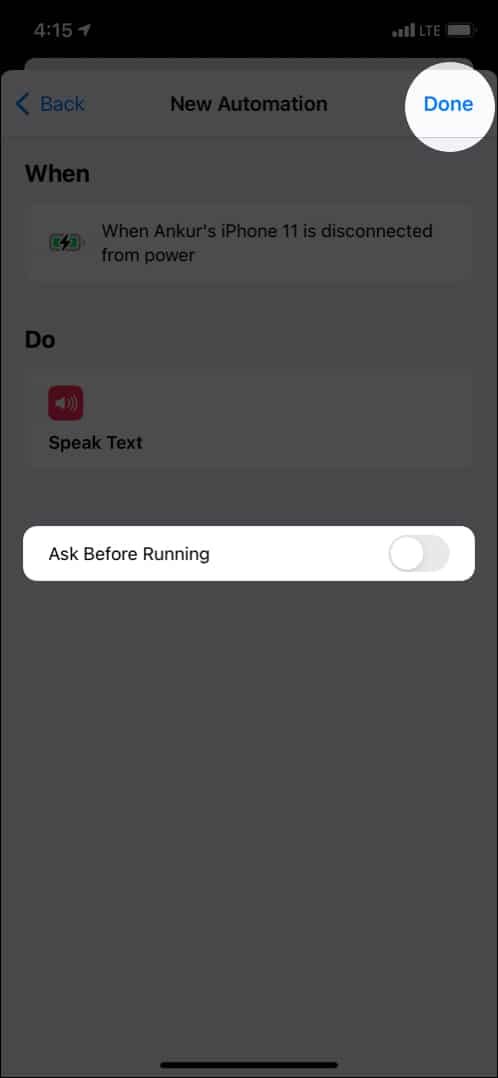A screenshot of a cell phone interface is displayed, containing multiple sections highlighted in white against a grayed-out background. At the top left corner, the time is shown as 4:15. In the top right corner, symbols indicate a fully charged battery, LTE connectivity, and full signal bars. Below these indicators, "Back" is written next to a blue left-pointing arrow.

Centered in the image, the text "New Automation" is prominently displayed in black, with the word "Done" written in blue inside a white circle. Beneath this header is a section labeled "When." This section features a horizontal green battery icon with a black lightning bolt, accompanied by the text, "When Ankur's iPhone 11 is disconnected from power." 

Following this, the word "Do" introduces another section, marked by a red square containing a speaker icon. Below this, in black text, is the command "Speak Text." Lastly, a white horizontal rectangle at the bottom includes the gray text "Ask Before Running." The entire layout is underscored by a three-inch horizontal black line at the bottom center of the image.